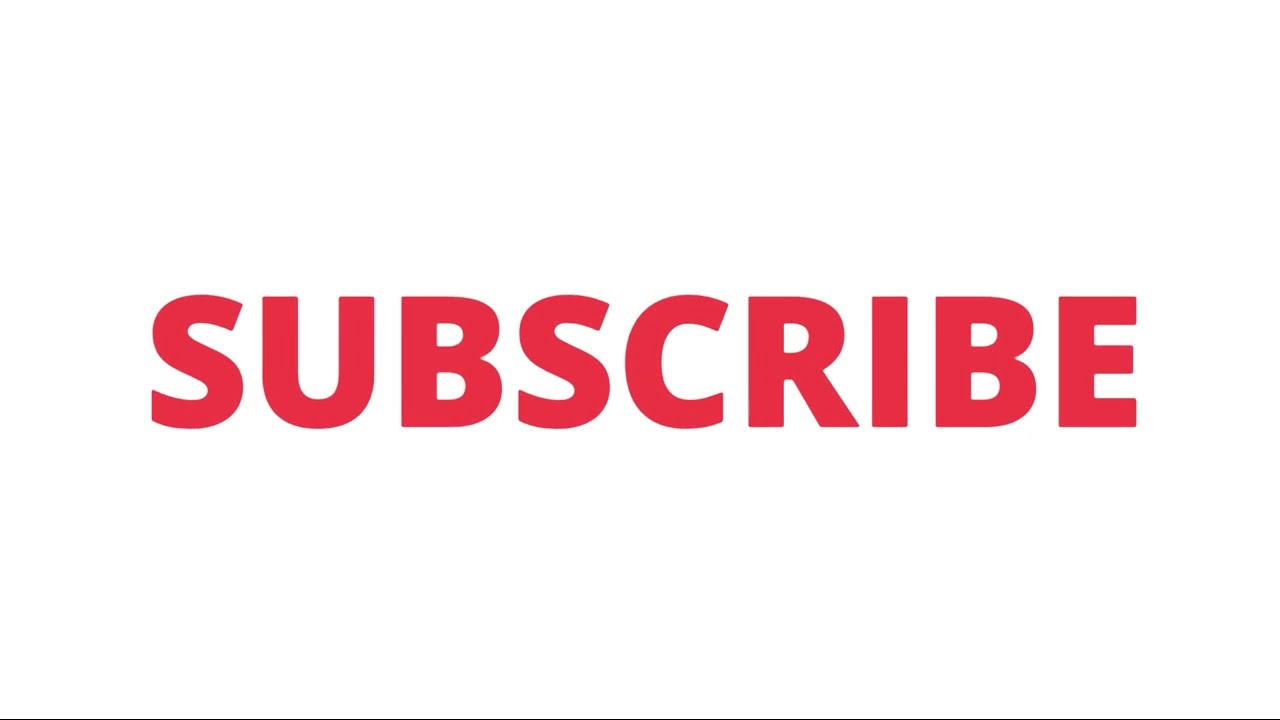The image is a horizontal rectangle with a white background, prominently featuring the word "SUBSCRIBE" in bold, capitalized, sans serif font. The lettering is a vibrant red, spanning from the left edge to the right edge of the image, positioned centrally. The image is of high clarity, with no blurriness or distortion. Below the red text, there is a narrow gray line running along the very bottom of the image. No other text, objects, or numbers are present, giving the image a clean and focused appearance.